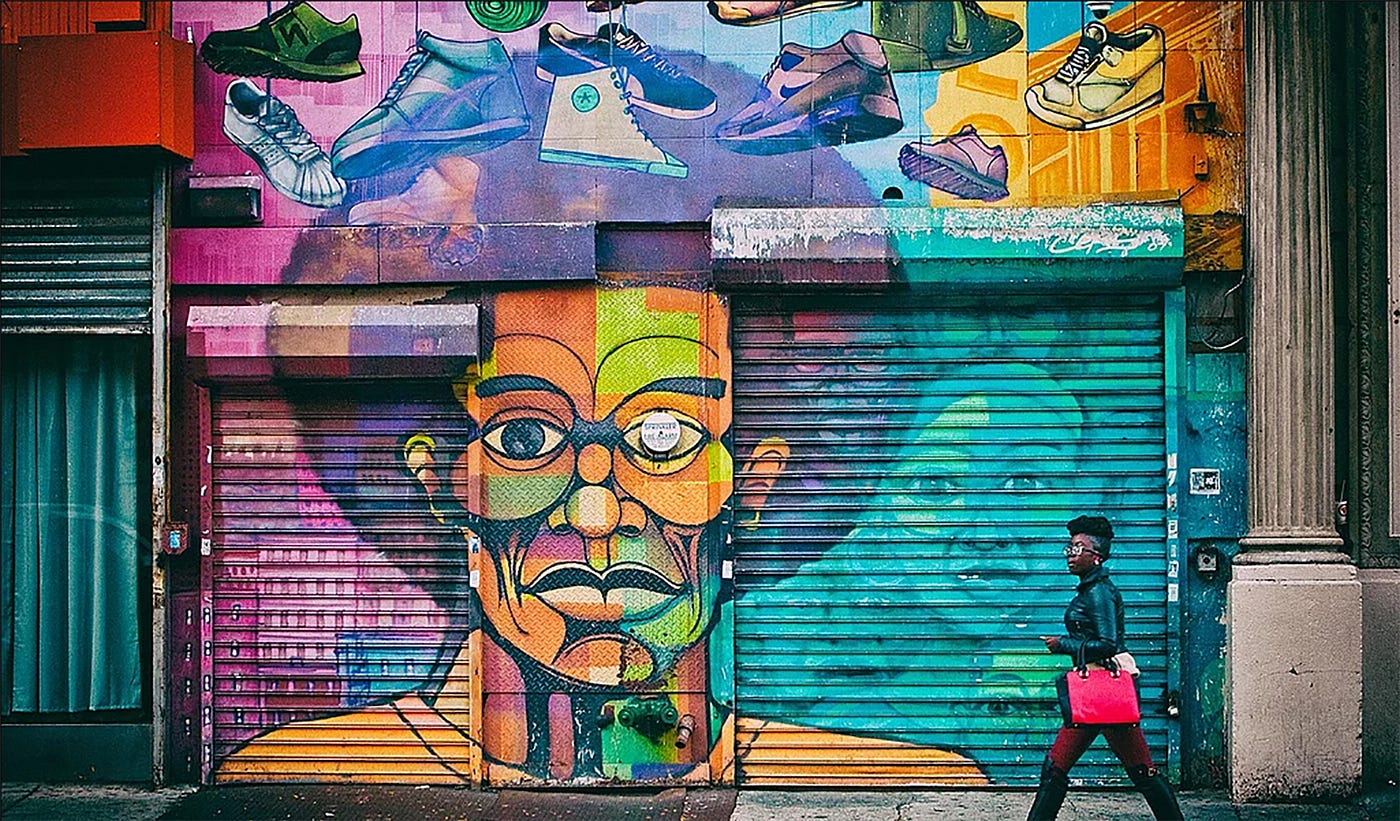A black woman, dressed in a stylish leather coat with maroon pants and black boots, walks along the street carrying a pink purse. She strolls past a vibrant and eye-catching mural painted on the exterior of a store. The mural features an African American man with an afro depicted in a mosaic style with vividly colored squares in hues of yellow, green, blue, and red, giving him a futuristic look. He appears to wear glasses, but closer inspection suggests he may not be. Above him, various painted tennis shoes—ranging from brands like Converse and Nike—hang in a spectrum of colors including white, black, blue, and purple, adding to the mural's colorful vibrancy. To the right, the mural extends to depict a woman's face in shades of blue and green. The overall scene is a burst of artistic expression, blending street fashion and urban art seamlessly.